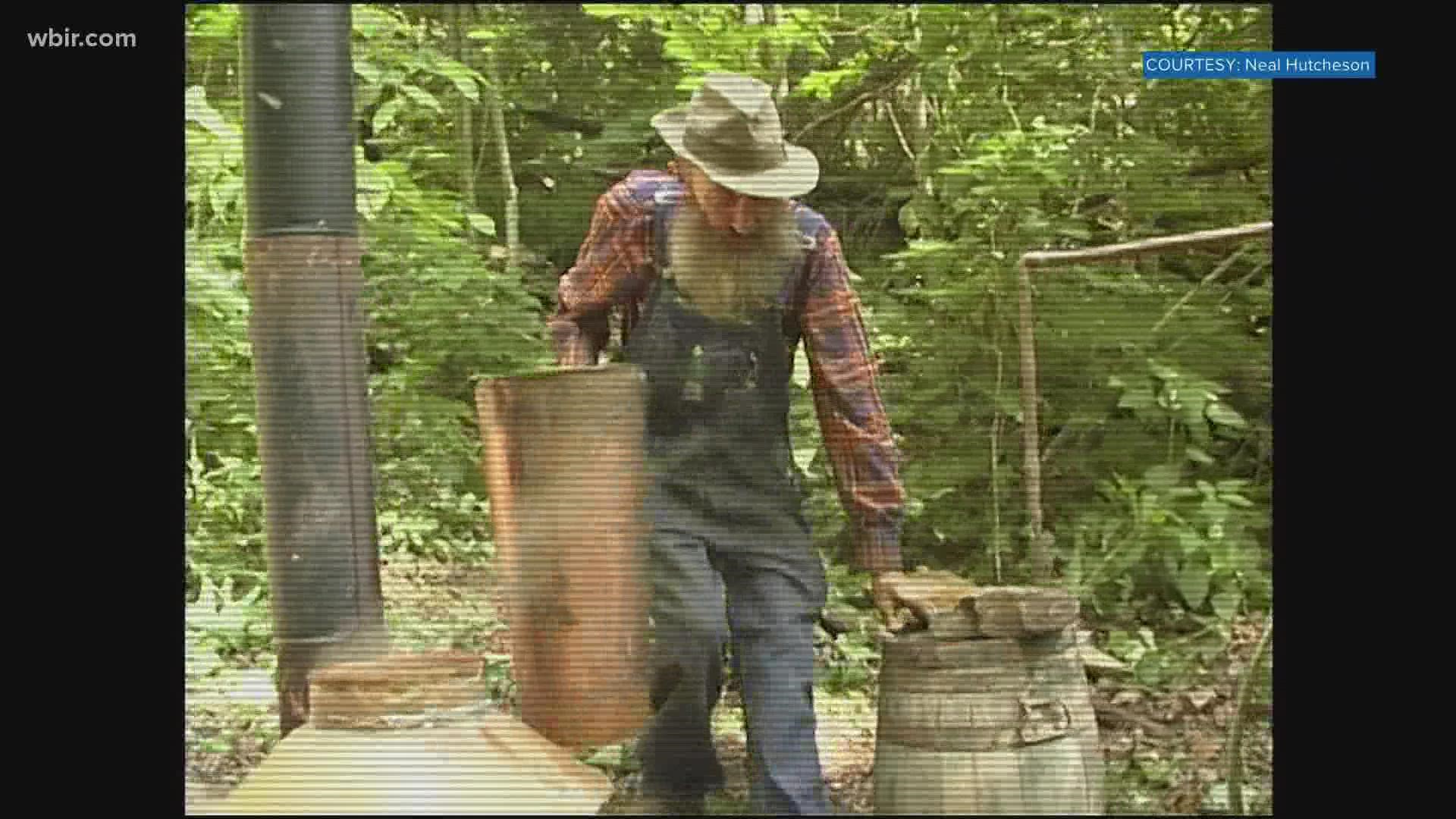In this screen capture taken from a TV screen, the image features an older man dressed in blue overalls and a red and blue long-sleeve shirt. He is wearing a beige fedora-style hat and sports a long gray beard that reaches down to his neck. The man appears to be performing some sort of chore, possibly related to brewing or farming, as he holds a small wooden barrel in his right arm. Next to him, there is a tin barrel and a long, segmented pipe or pail that is brown and black, suggesting the setup may be for making a liquid or smoking process. The background is verdant with green trees and leaves, indicating the setting is outdoors during the daytime. Text overlays in the top corners of the image reveal the website WBIR.com on the left and "Courtesy Neil Hutchison" in a blue rectangle on the right.